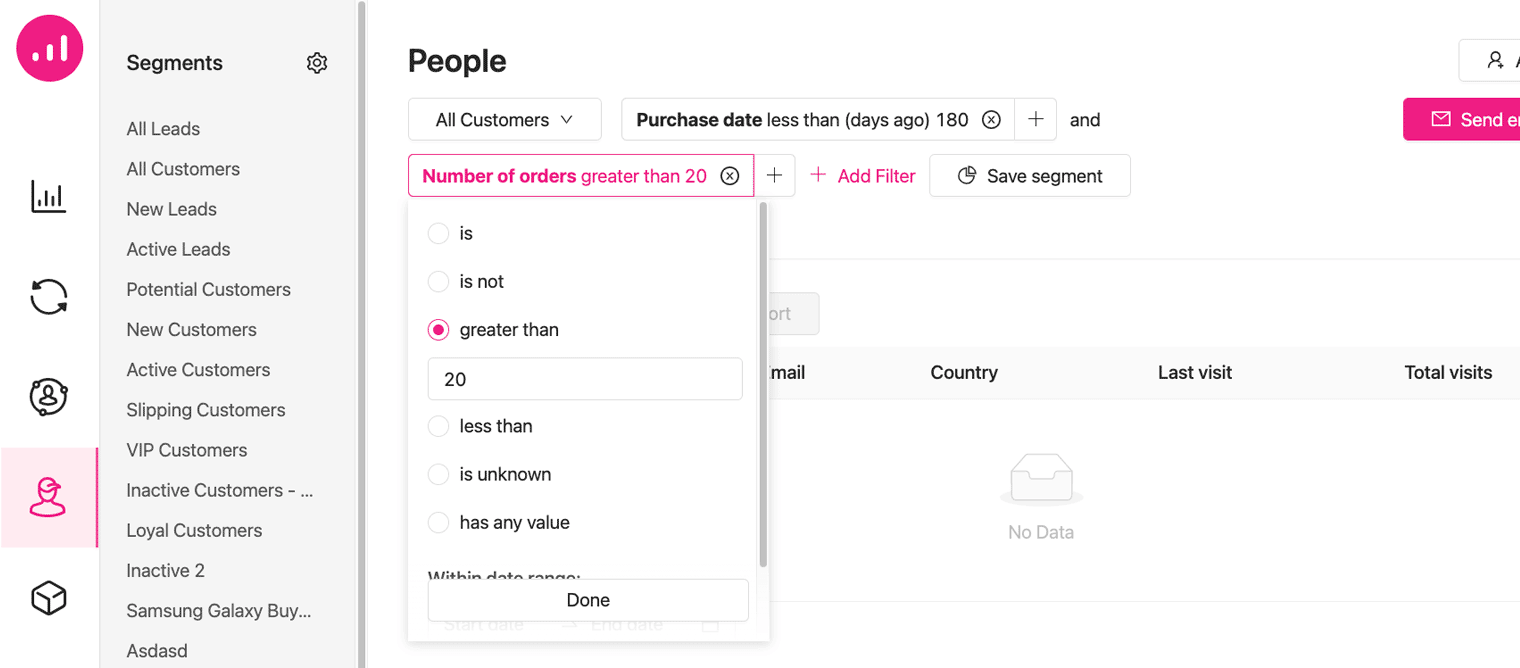The image depicts a web page with a complex layout and various interactive elements designed for managing customer data. On the left side of the page, there is a vertically aligned navigation bar featuring several icons: 

1. A purple-pink circle with three rising bars representing a graph.
2. Another graph icon.
3. Two circular arrow icons.
4. A small person icon.
5. A pink-highlighted icon of a person wearing a hat.
6. A 3D cube icon. 

Following this, the page transitions into a gray section containing another vertical navigation bar with multiple entries:
- Segments
- A cog icon (likely settings)
- All Leads
- All Customers
- New Leads
- Active Leads
- Potential Customers
- New Customers
- Active Customers
- Slipping Customers
- VIP Customers
- Inactive Customers
- Loyal Customers
- An entry labeled "Samsung Galaxy" with trailing ellipses (“Buy...”)
- An entry named "ASDASD"

To the right of these navigation bars, another part of the page displays the following content:
- A section labeled "People."
- A dropdown menu titled "All Customers."
- A dropdown labeled "Purchase Date" with the condition "less than (days ago) 180," alongside an "X" button and a "+" sign.
- Another dropdown highlighted in purple reads "Number of orders greater than 20" with an "X" button and a "+" icon.
- A pink "Add Filter" button.
- A "Save Segment" tab.
  
Below the "Number of orders greater than 20" dropdown, there are additional filter options:
1. Is
2. Is Not
3. Greater Than (selected with a pink dot and filled with the value 20)
4. Less Than
5. Is Unknown
6. Has Any Value

A "Done" button is situated to the right of these options.

Further to the right, partially covered tabs include:
- Mail
- Country
- Last Visit
- Total Visits

Beneath these tabs is an empty mailbox icon with the label "No Data."